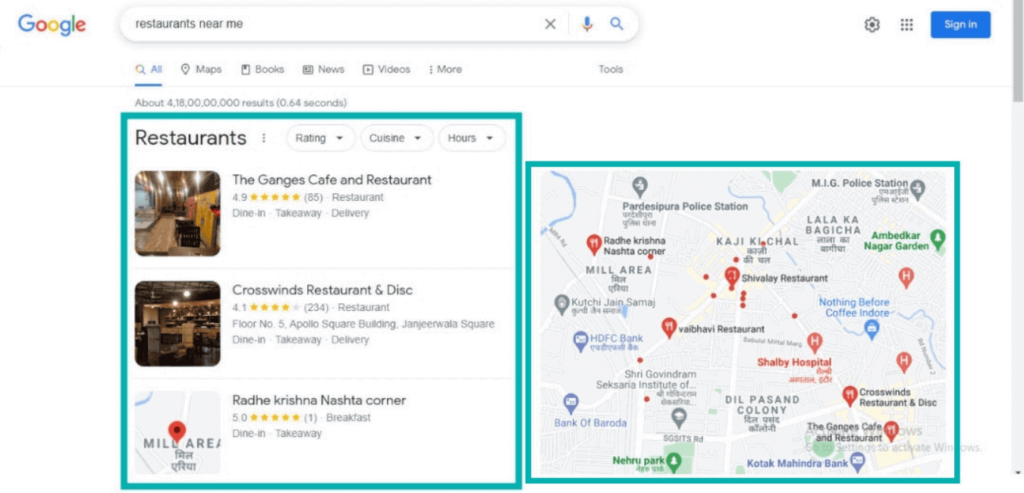This detailed caption describes a Google search results page specifically focused on finding nearby restaurants:

---

The image features a Google search results page with a white background. At the top left corner, the vibrant Google logo is prominently displayed in its iconic colors: blue, red, yellow, blue, and red. Adjacent to the logo is a search bar with the query "restaurants near me" entered. To the immediate right of the search bar, there's a gray 'X' for clearing the query, followed by a microphone icon for voice search, and a blue search icon to initiate the search.

Extending to the right of the search bar, a navigation menu offers various search options including "All," "Maps," "Books," "News," "Videos," and "More." At the top right corner of the page, a blue "Sign in" button invites users to log in.

Below the search bar, a section outlined in blue displays snippets of restaurant search results. The first snippet is highlighted, presenting "Orangest Cafe and Restaurant" with an accompanying interior image. The restaurant boasts a rating of 4.9 stars. Following this, the "Crosswinds Restaurant and Desk" is listed with a 4.1-star rating. Below these listings, a map with a red location pin is shown.

To the right of these snippets, another restaurant, "Ratee Christina Nashta Corner," is prominently displayed with a commendable 5-star rating. Adjacent to this, a blue-outlined square contains a map featuring multiple pins in red, blue, and green, indicating various restaurant locations.

---